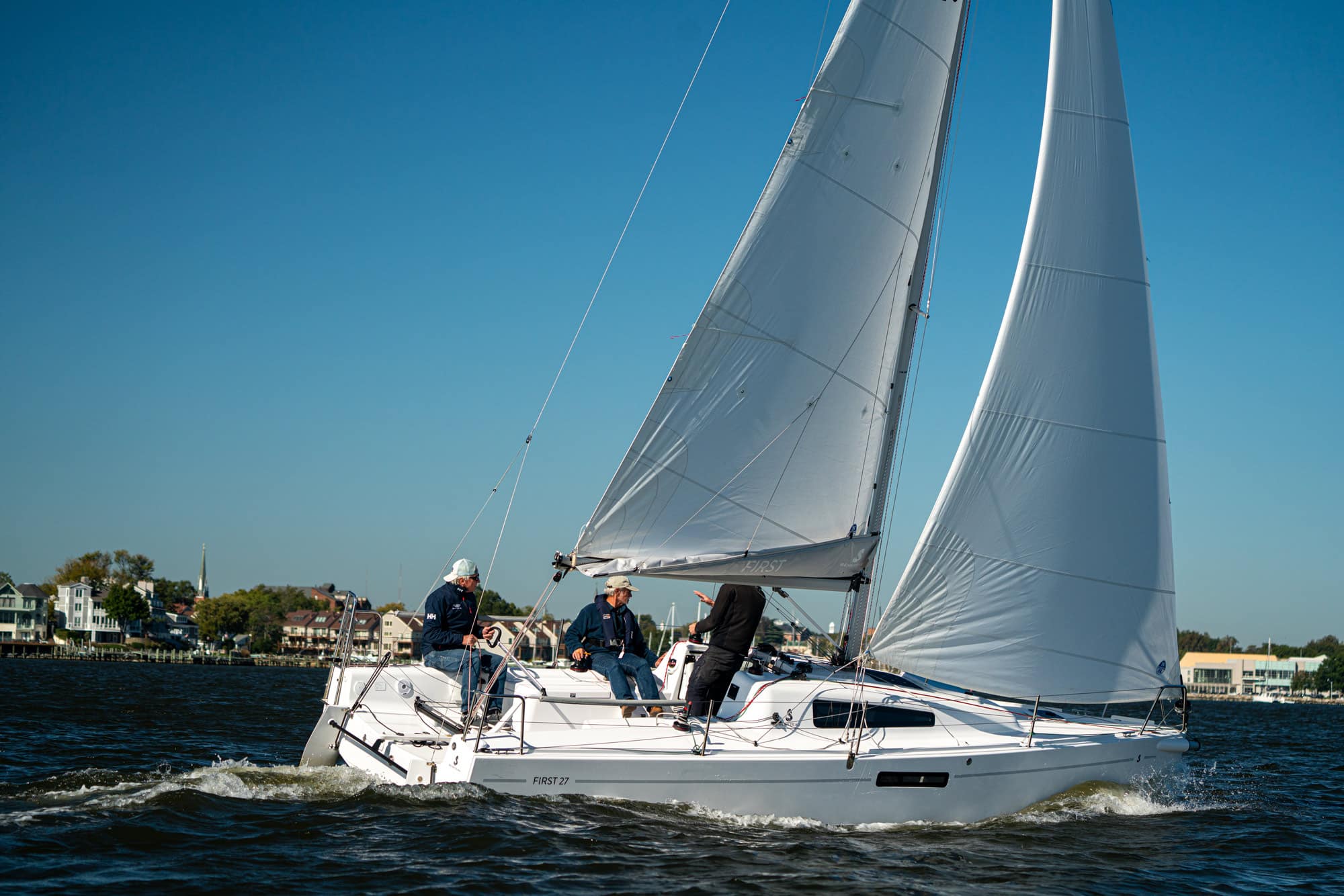The photograph captures a serene day at a marina, featuring a sizable white sailboat with two fully hoisted white sails. Onboard, there are three crew members dressed in long-sleeved shirts and jeans, indicative of cooler weather. Two crew members are visible, facing the camera, wearing backward white hats, blue jackets, and blue jeans. The third person, whose face is not visible, is standing with his back to the camera, dressed entirely in black. The boat appears to be moving smoothly through calm waters, leaving ripples behind. Small windows peek just above the waterline of the boat. In the background, a mix of beach houses or condos, fences, and green trees lines the distant shore. The sky above is a clear, vivid blue, free of clouds, complementing the tranquil marine setting.